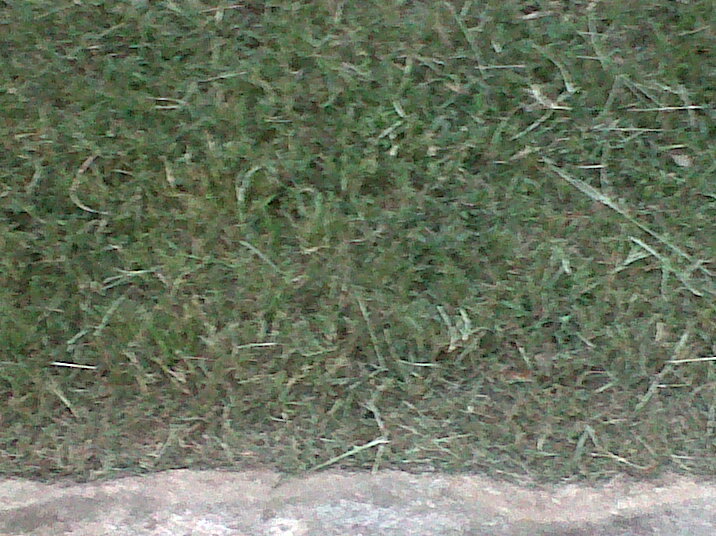The image depicts a small patch of predominantly green grass, speckled with patches of white and brownish-yellow blades, indicating some grass may be dying or dried out. The grassy area covers most of the image, approximately 90% of it. At the bottom of the image, there is a grayish portion, possibly the edge of a sidewalk, a piece of stone, or cement, which could suggest this patch of grass is adjacent to a man-made structure. The generally bright lighting suggests it was taken during the daytime, though the image is somewhat blurry, possibly due to a hazy effect or minor distortion. The photo captures the mixed state of the grass, with some blades looking fresh and green, while others are white and dried out, potentially from recent mowing or lack of water.